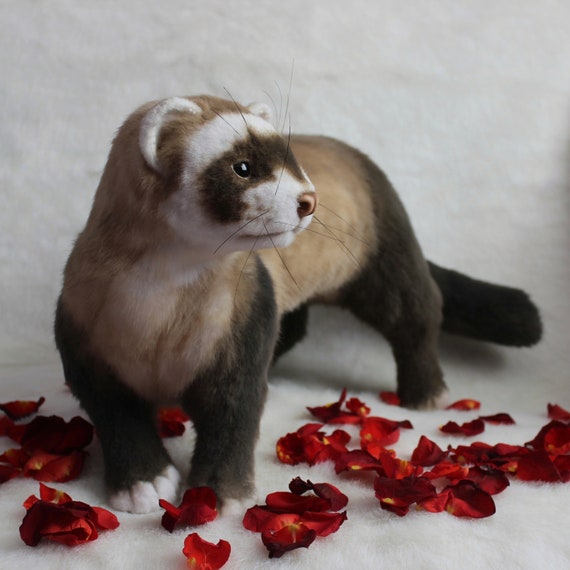This is a detailed, square-format color photograph of a stuffed ferret toy or a real-looking taxidermied animal. The creature resembles a weasel or stout with distinct markings: it has a long, light brown body, a light brown torso, and dark brown fur on its short legs and hind legs. Its face features a white color with a dark brown mask across its eyes and is adorned with long whiskers. The ears have white edges, and the toy has a calm expression, gazing toward the right side of the image. The animal is placed on a fluffy white surface, reminiscent of a white fur carpet, against a white background. Scattered around the surface are red rose petals, adding a contrasting splash of color to the scene.